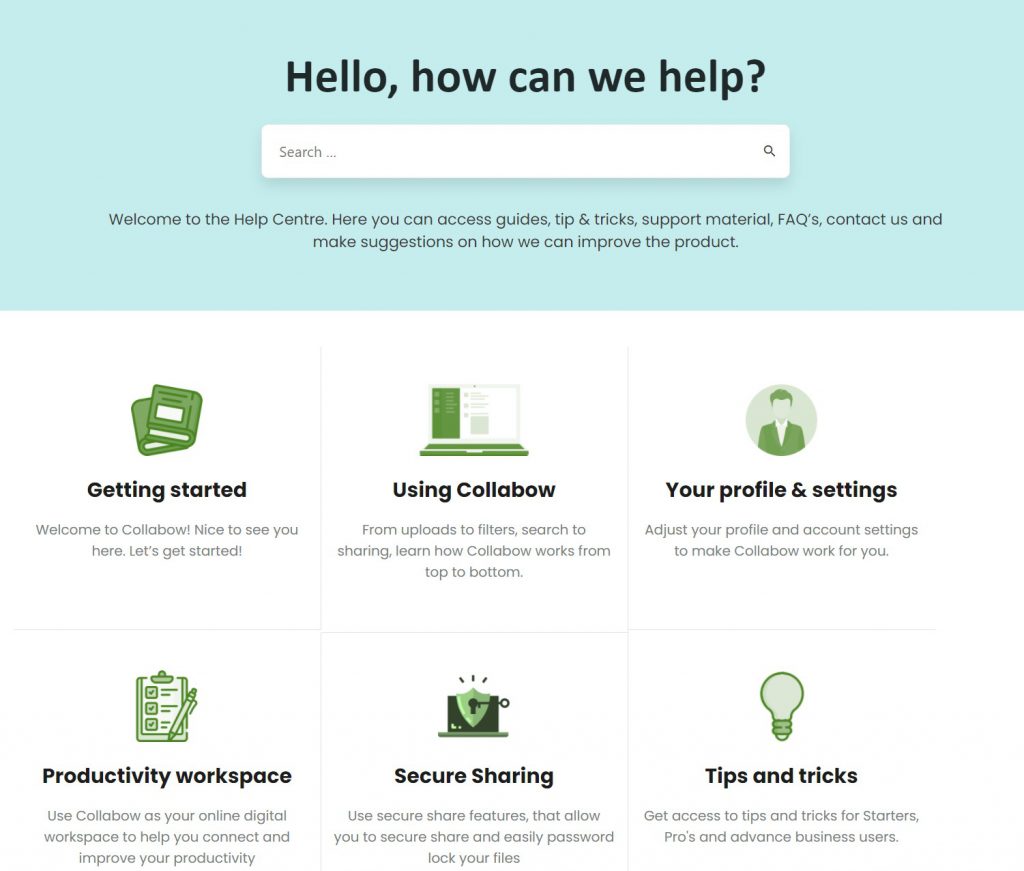This is a photograph capturing a web page with a prominently featured blue header at the top, adorned with the greeting, "Hello, how can we help?" Immediately below the header, there is a search field characterized by a large drop shadow and a small magnifying glass icon on the right. The placeholder text within the search bar reads, "Search..." 

Beneath the blue header, there's a welcoming message: "Welcome to the Help Center." This section elaborates that users can access a variety of resources including guides, tips, tricks, support materials, FAQs, contact options, and suggestions for product improvement.

Six sections are organized below this introduction, displayed in a three-by-two grid. Each section is marked by a header accompanied by an icon in green and gray, along with detailed text explaining the contents:

1. **Getting Started** - Represented by two book icons, this section is about starting to use the service.
2. **Your Profile and Settings** - Illustrated with an icon of a person within a circle, this section guides users on adjusting their profile and account settings.
3. **Productivity Workspace** - Denoted by a clipboard icon, this section focuses on enhancing productivity.
4. **Secure Sharing** - Marked by a shield with a key icon, this section addresses security and sharing elements.
5. **Tips and Tricks** - Illustrated with a light bulb icon, this section offers various tips and tricks.

The detailed text beneath each section is in gray, providing deeper insights into each area. For example, under "Getting Started," the text reads, "Welcome to Colabo, nice to see you here! Let's get started." It further explains topics such as uploads, filters, search capabilities, and sharing functionalities. 

Overall, the web page presents itself as a generic, templated Help Center, designed to assist users with various aspects of using the Colabo platform.